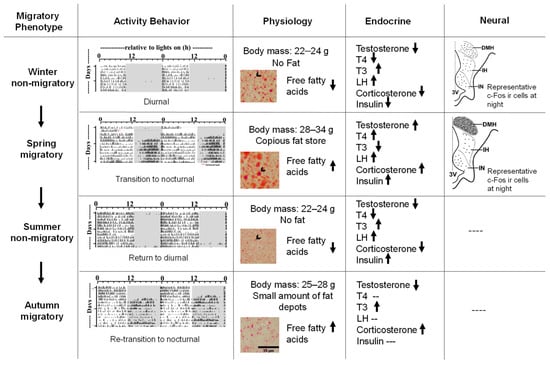This detailed landscape-oriented infographic chart illustrates the various phases of the migratory phenotype across seasons, focusing on winter non-migratory, spring migratory, summer non-migratory, and autumn migratory stages. The x-axis at the top features four main columns: Activity Behavior, Physiology, Endocrine, and Neural.

In the Activity Behavior column, smaller sub-charts illustrate the transition of activity patterns: diurnal activities in winter, shifting to nocturnal in spring, reverting to diurnal in summer, and transitioning back to nocturnal in autumn.

The Physiology column provides data on body mass fluctuations and fat changes for each season, represented within tan squares dotted with red markers.

The Endocrine column is detailed with arrows indicating fluctuations in hormones such as testosterone, T4, T3, LH, corticosterone, and insulin, showcasing their increase or decrease during different seasons.

In the Neural column, there are diagrams only for the winter non-migratory and spring migratory phases, indicating representative CFOS cell activity at night, captured through grayscale images.

Overall, this chart comprehensively captures the seasonal changes in migratory phenotype activity behaviors, physiological metrics, hormonal levels, and neural representations.